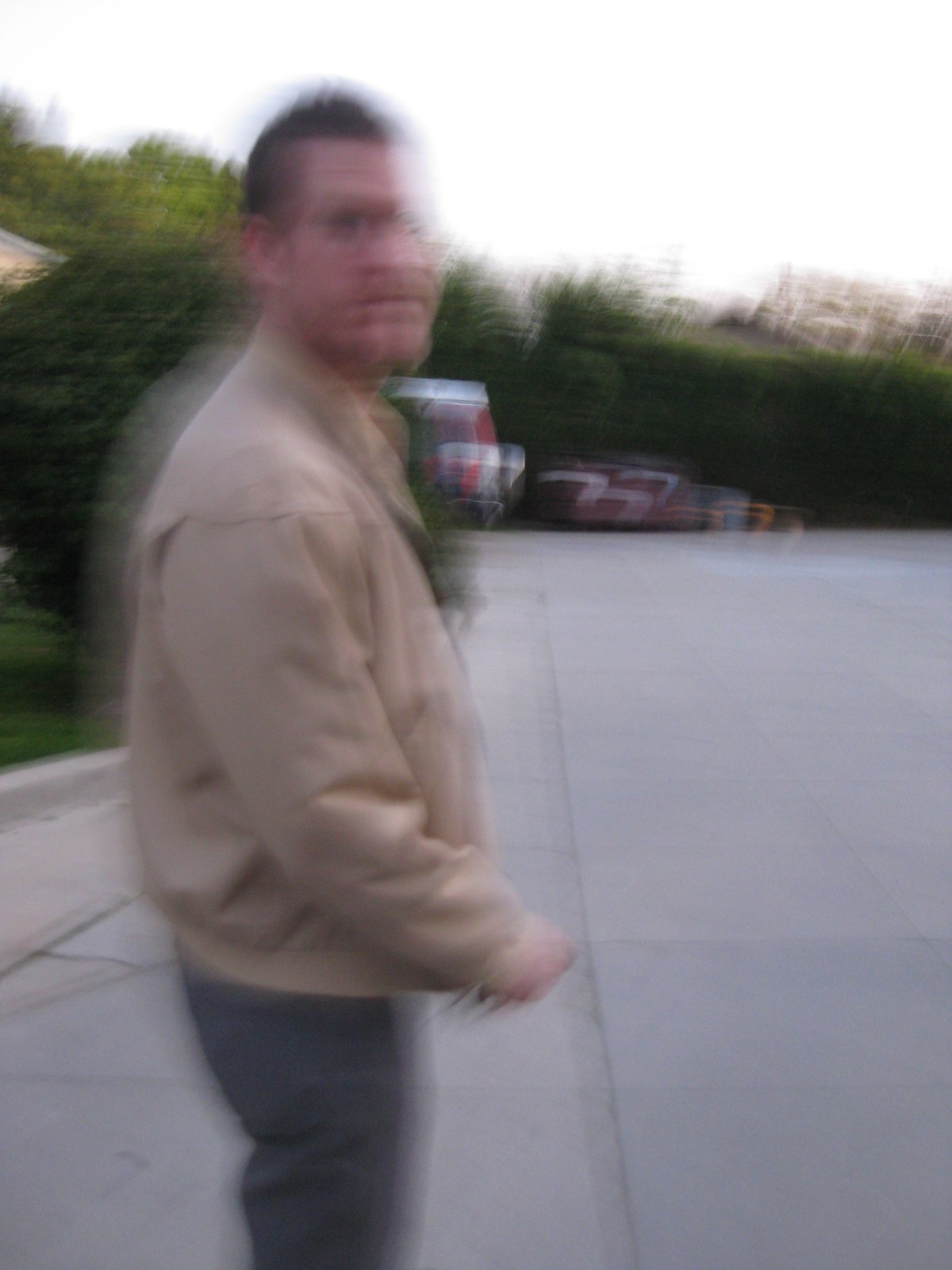In this extremely blurry image, there appears to be a man dressed in gray pants and a tan-colored jacket. He is holding an indistinct object in his right hand and has just turned to glance toward the camera, giving the impression that he is on the move. The man, who is likely Caucasian, has dark brown, very short hair and seems to have a faint mustache and beard, though the image's blurriness makes these details hard to confirm. He is standing in a large concrete parking lot, which extends into the background. There are some vague, squiggly shapes that might be a car, situated further back in the parking lot. Surrounding the lot on the left side and extending into the distance is a dense array of trees in full bloom, displaying a mix of dark and medium green foliage.